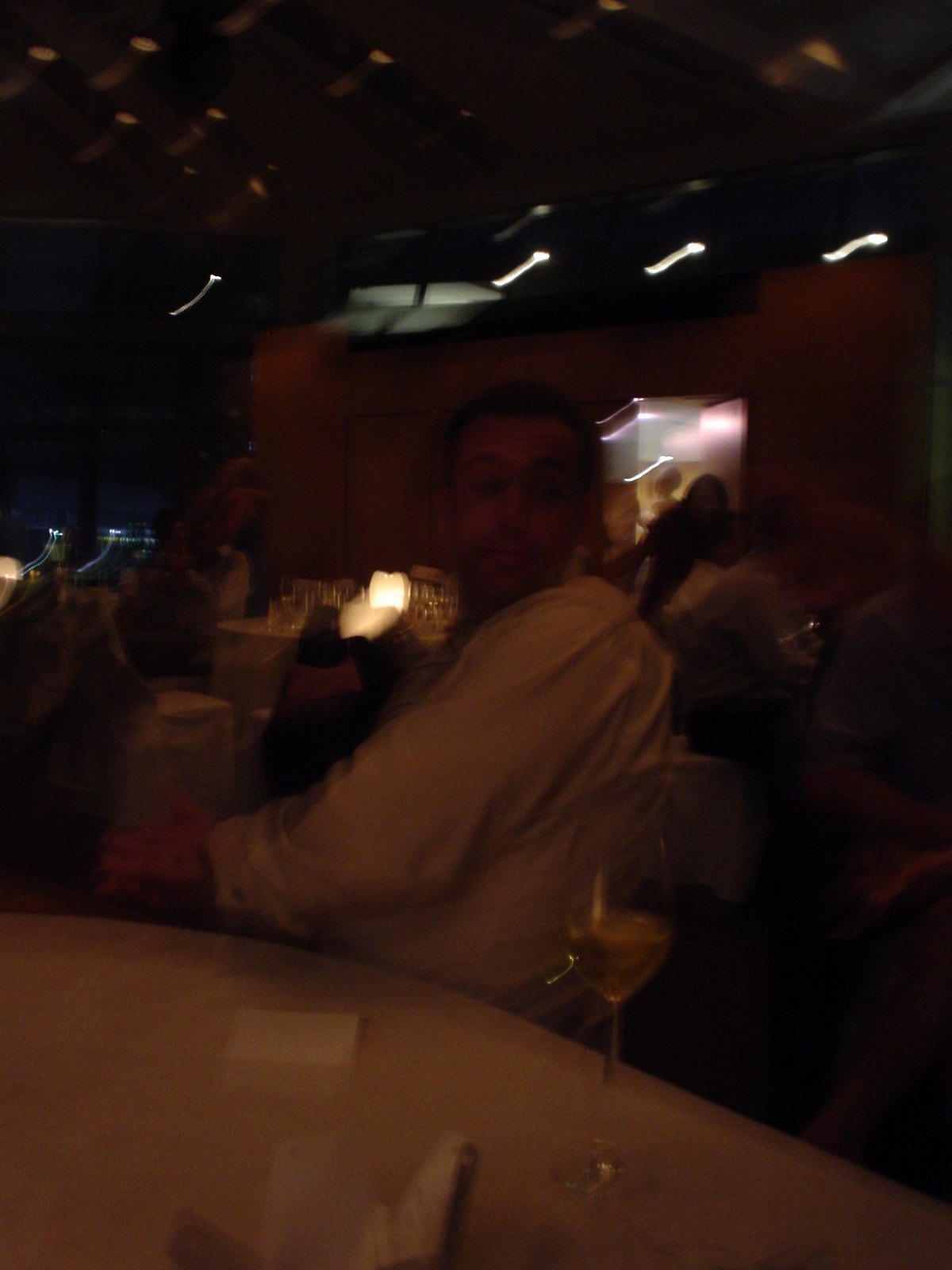The color photograph, taken indoors in a lounge bar, captures the ambiance in low light with a blurred effect, likely due to a long exposure and camera movement. The lighting, featuring both white and yellow hues, appears as elongated streaks across the ceiling, adding a dynamic sense of motion to the image. 

In the center lower half of the photograph, the main subject—a man in a long-sleeved shirt adorned with a cufflink on his left sleeve—dominates the scene. On his right, a drink rests on what appears to be a bar or table. 

To the back right, an open metallic door stands out due to its stark lighting, contrasting sharply with the otherwise dim environment. Through the door, a figure is visible, hinting at activity beyond the lounge. 

In the background, to the left of the man whose head is turned towards the camera, a small table lamp or similar illumination adds a cozy but slightly obscured detail typical in a lounge bar or comedy club setting.